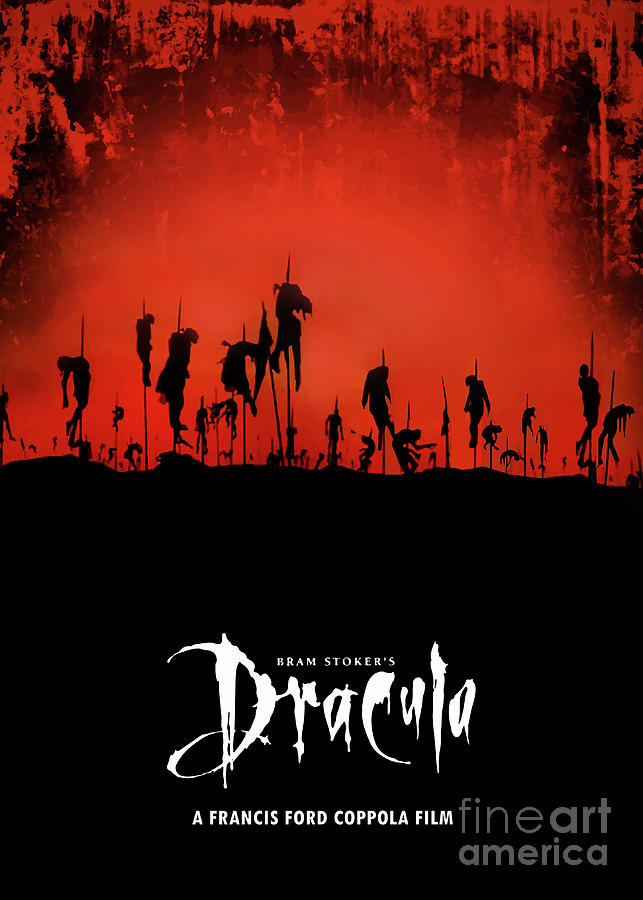This movie poster for "Bram Stoker's Dracula," directed by Francis Ford Coppola, is visually striking and unsettling. The upper part of the image is a vivid, bright red background with some black shadowy brush strokes swirling ominously near the top. Dominating the top half is the impression of blood-smeared paint, creating an eerie and menacing atmosphere.

The bottom half of the poster is dominated by a silhouette of a solid black hill. Within this hill, the stark black forms the base for disturbing imagery. Silhouetted against this dark expanse are the haunting outlines of numerous impaled figures. There are at least 18 clearly defined people, cruelly mounted on sharp stakes. The stakes thrust high, displaying individuals in various distressed poses—some with stakes driven vertically through their bodies, others bent forward agonizingly.

At the very base of this grim scene, in bold white text, the title "Bram Stoker's Dracula" is prominently displayed, with the word "Dracula" appearing as if it were painted in blood. Below this, it reads "a Francis Ford Coppola film" in elegant print. In the bottom right corner, a small, unobtrusive gray watermark for Fine Art America confirms the source of the artwork. This poster starkly captures the dark intensity of the classic horror story.